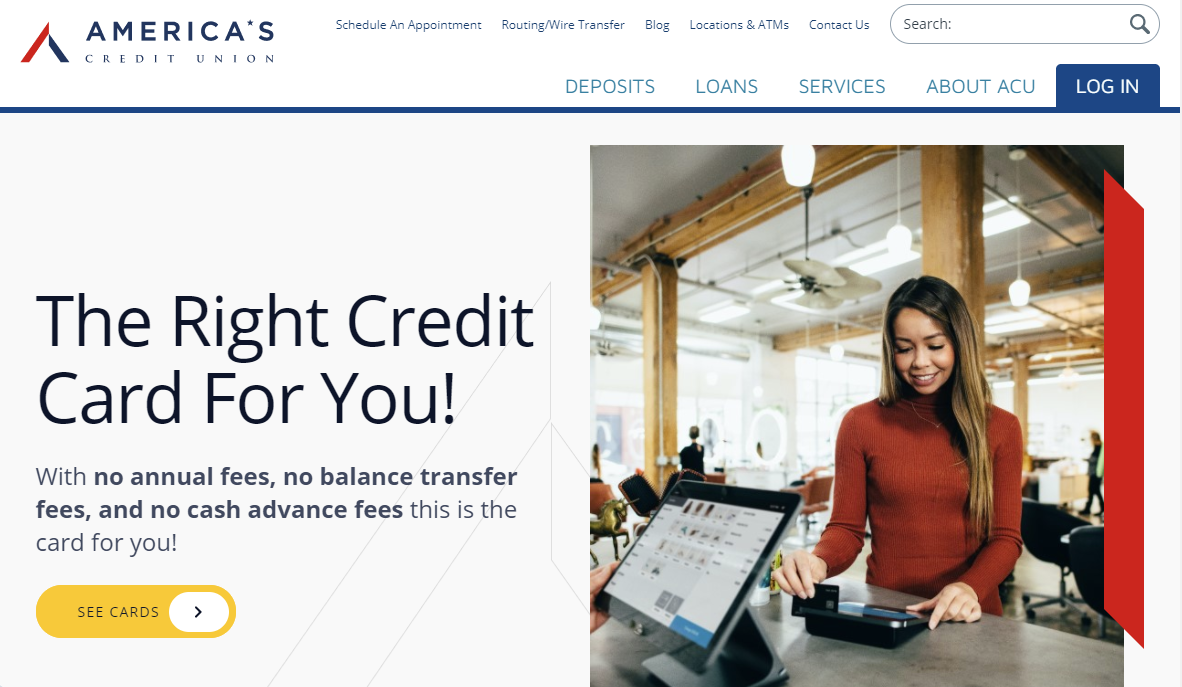The homepage for America's Credit Union features a well-organized layout. At the top of the screen, five tabs read "Schedule an Appointment," "Routing or Wire Transfer," "Blog," "Locations and ATMs," and "Contact Us." In the top right corner, there's a search bar with the word "Search" and an accompanying magnifying glass icon. 

Beneath this navigation header, five larger tabs are arranged from left to right: "Login" (which is currently highlighted), "About ACU," "Services," "Loans," and "Deposits." 

Dominating the right side of the screen is an inviting image of a woman in a spacious, high-ceilinged area featuring wooden columns and exposed wooden beams. Large storefront windows flood the space with natural light. The woman, dressed in a brown turtleneck sweater, with long light brown hair cascading down, is standing at a counter. She's in the process of swiping her card on a tablet reader and is smiling down at the device as she completes this task.

Complementing this welcoming scene, the left side of the screen displays the phrase: "The right credit card for you."